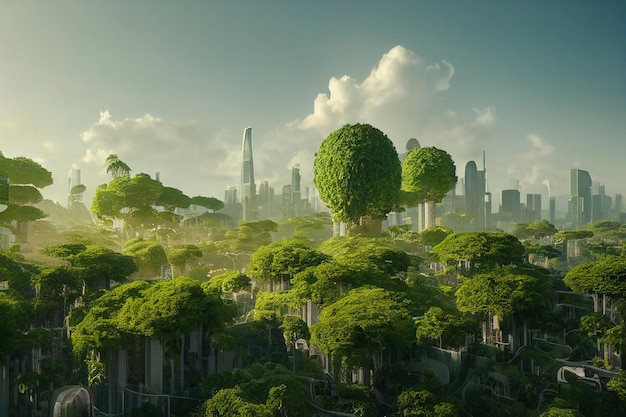The image presents a richly detailed futuristic cityscape where nature and industry coexist in an intriguing harmony. In the foreground, a verdant layer of vegetation, featuring green vines and tall trees with circular tops, drapes over pristine white structures, suggesting nature's reclamation of the urban environment. The vegetation is lush and vibrant, starkly contrasting with the metallic and modern aesthetic of the city. Amidst the foreground greenery, paths seem to wind through the leafy landscape, hinting at a possible symbiotic relationship between nature and human infrastructure.

Dominating the middle of the scene, a uniquely spherical tree stands tall, capturing attention with its prominence. Beyond this lush foreground, a series of modern buildings and skyscrapers, tinged with a subtle green hue, rise majestically into a sky painted with fluffy white clouds. The tallest skyscraper, slightly left of center, features an arched top and towers over the cityscape, adding an element of grandeur.

The background continues to tell the tale of this blending of green and urban, with a clear blue sky that transitions into a gentle fog, shrouding the distant skyline in mystery. The greenish cast to the entire image gives it an otherworldly quality, further enhancing the dreamlike vision of a future where nature and humanity seamlessly blend together.